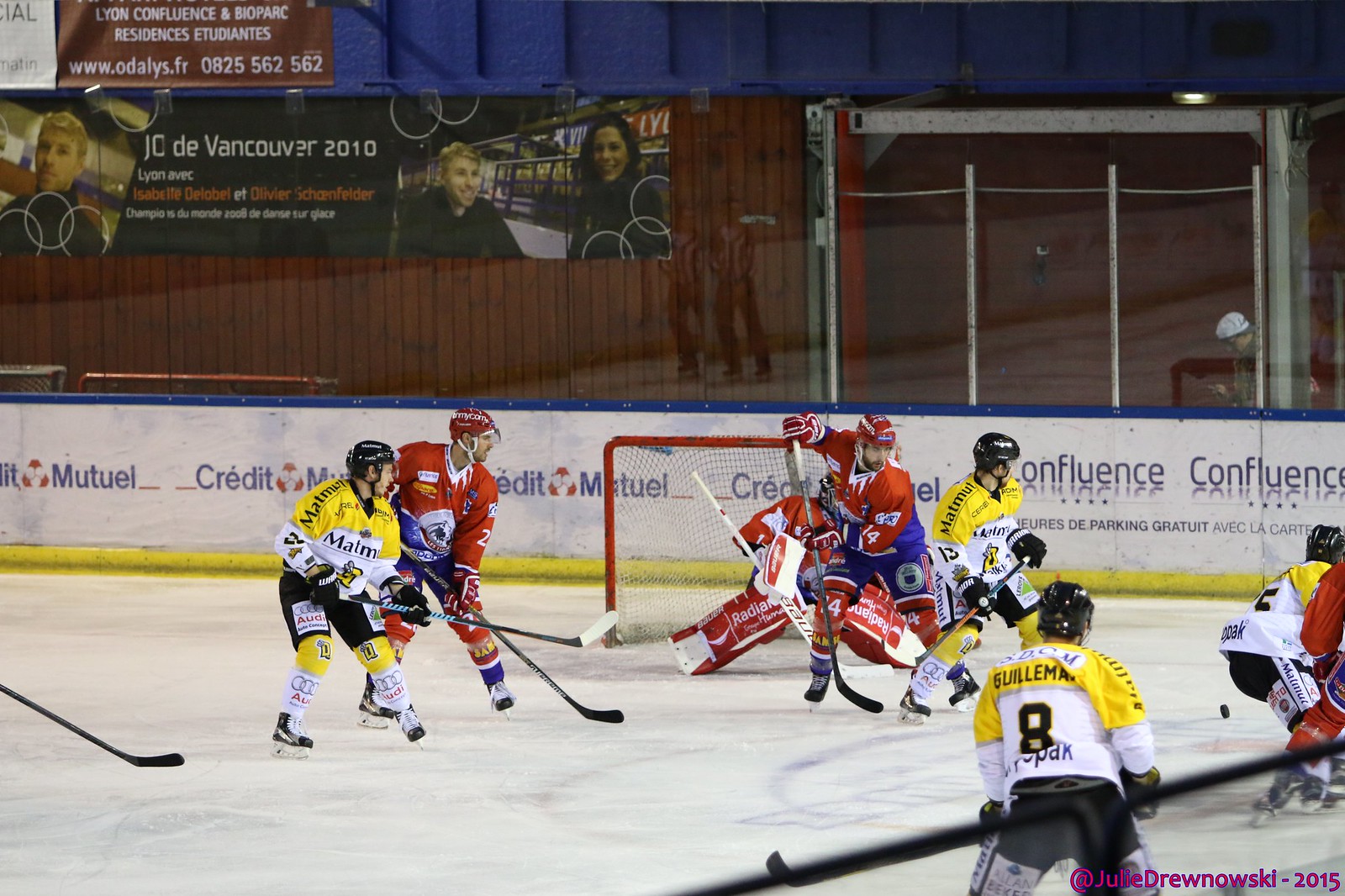The image captures an intense moment of a hockey match at a rink, possibly indoors. It shows two teams in vibrant, contrasting uniforms: the red team, donned in red jerseys with blue shorts, red chin protectors, and red helmets, positioned defensively around their red-framed goal. The opposing team, dressed in yellow and white jerseys with black shorts and helmets, is on the offensive, with player number 8 noticeably visible. Three yellow team players are actively engaged in passing the puck, while the red team's goalie, fully alert, tracks the puck to protect the goal. The background shows glass partitions, likely separating the rink from the audience area, though no spectators are discernible. Above the partitions, a banner advertises the sponsors, "Credit Mutuel" and "Confluence," reflecting a French connection. A watermark at the bottom credits the photo to Julie Drunowski, 2015.